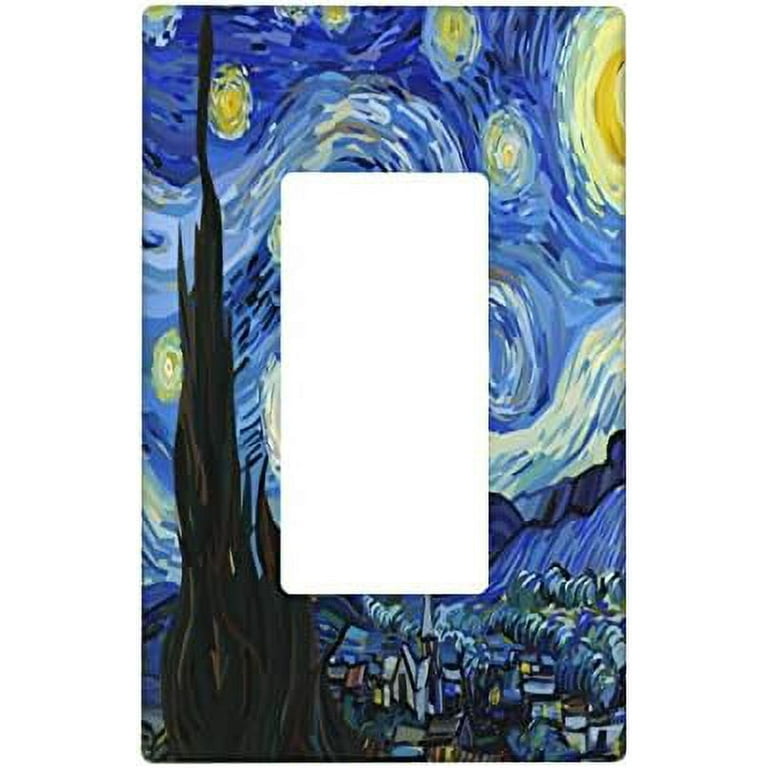This image is a modified version of the famous painting "Starry Night" by Vincent van Gogh. The vertical, rectangular painting features a large, white rectangular cutout in the center, resembling a cell phone shape or photo frame. Surrounding this cutout, the iconic dark blue swirling night sky, accented with vibrant yellow stars and a partially visible moon, is prominently displayed. The town below, complete with distinct structures such as a church, is bathed in the cool hues typical of van Gogh's palette. A tall, dark brown cypress tree, devoid of leaves, dominates the left side of the image. This alteration disrupts the painting's famous celestial swirls while the serene town beneath remains almost fully visible.